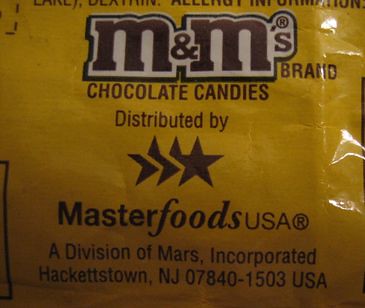This image features a close-up of an M&M candy prominently displaying its branding. The candy is yellow, appearing somewhat dark due to low lighting conditions, which gives it a richer, darker hue. The surface of the M&M is characteristically plastic-like with a slight wrinkling on one side that catches and reflects light, giving it a distinctive sheen.

At the top of the candy, the iconic M&M's logo is visible. This logo is crafted in brown text, set against a white background with a black border. Below this, in brown text directly on the yellow background, the inscription reads: "M&M's brand chocolate candies distributed by." Below this inscription, three interconnected five-point stars occupy a central position. Further down, the text continues: "Master Foods USA, a division of Mars Incorporated, Hackettstown, New Jersey 07840-1503 USA." The detailed branding and distribution information highlight the candy's authenticity and origin.